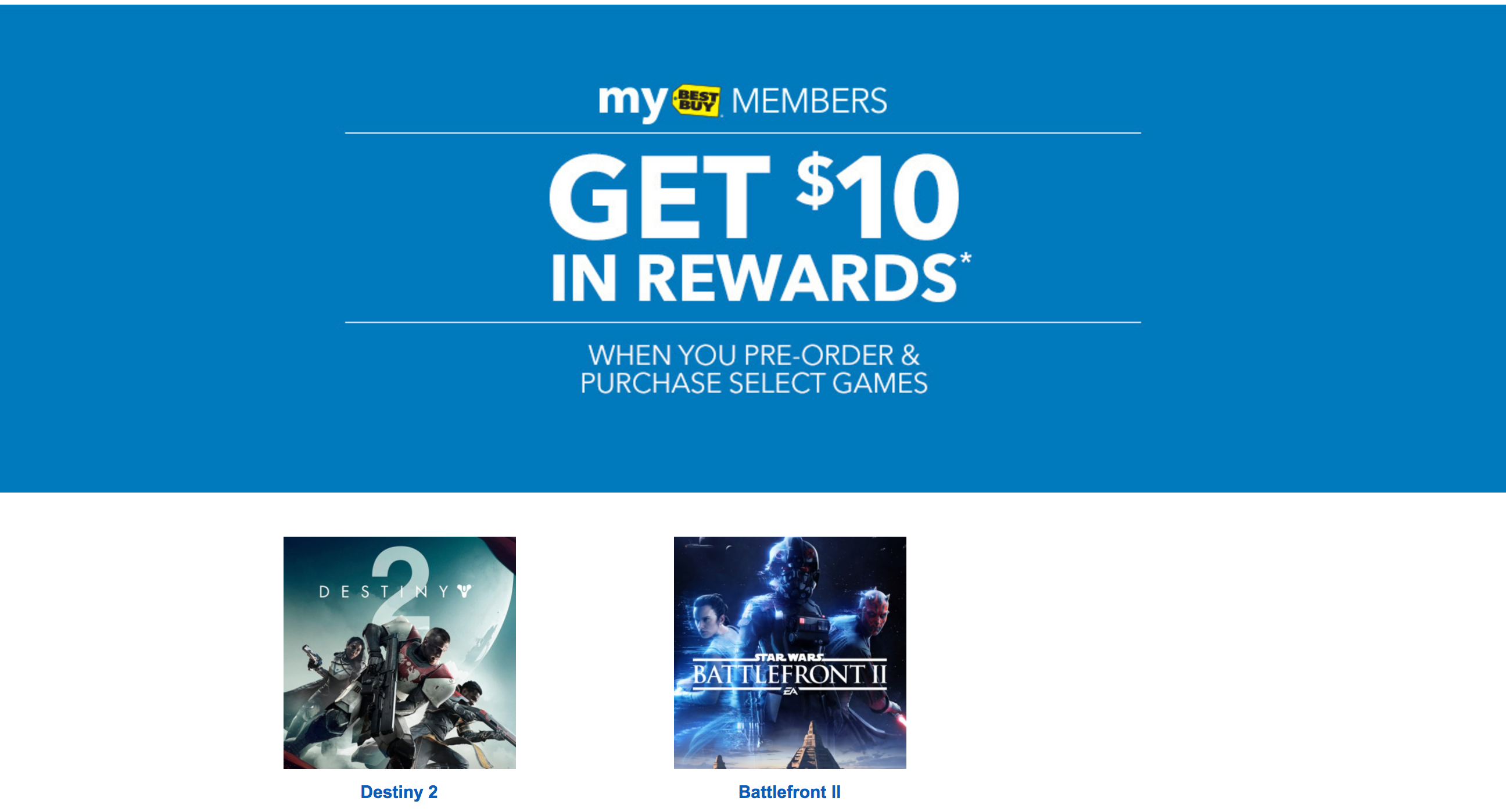The image is an advertisement divided into two distinct sections by color, with the upper section featuring a white background that transitions into a blue background. In the middle of the blue portion, centered vertically, white text reads "MY." To the right of this text is a yellow shopping tag icon adorned with black, all-caps text that reads "BEST BUY," with "BEST" on top and "BUY" beneath. To the right of the tag icon, thin white text spells out "MEMBERS."

Below this heading is a thin horizontal white line that extends roughly halfway across the width of the ad. Directly beneath this line, large white text declares "GET $10 IN REWARDS*". Another thin white line is positioned underneath this statement.

Beneath the second white line, small, tightly spaced, all-caps white text in two lines states "WHEN YOU PRE-ORDER AND PURCHASE SELECT GAMES," where the word "AND" appears as an ampersand ("&").

Switching to the white background section at the bottom, there are two square icons, each labeled with blue text beneath. The first icon, slightly bluish, features translucent white text reading "DESTINY" at the top. Behind this text is a large numeral "2." Positioned to the right of the "DESTINY" text is a white icon resembling a fidget spinner. Below this, three characters are depicted holding guns. The blue text beneath this icon identifies it as "DESTINY."

To the right, the second square icon primarily showcases a blue and black color scheme with three characters portrayed. Superimposed over these characters is a white title in a serif font that reads "BATTLEFRONT 2," accentuated by thin white lines above and below the title. The blue text label beneath this icon states "BATTLEFRONT 2."